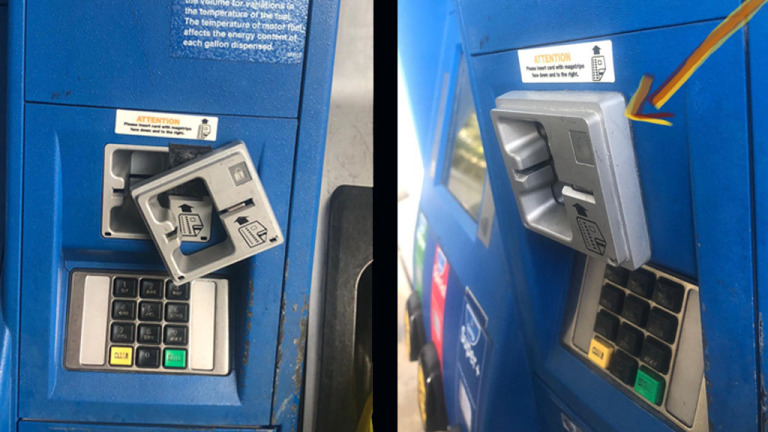This horizontally aligned photograph is composed of two side-by-side images of a blue fuel dispensing machine, separated by a black vertical line about a centimeter thick. Both images illustrate different angles of the same machine, with the left photo taken head-on and the right photo slightly angled.

In the left image, the main focus lies on a blue fuel dispenser with a black background extending from the top left to about three inches from the bottom. The photo captures details of the tampered card reader, which hangs off diagonally to the right, partially exposing its internal components. Above it, a white sign with mixed uppercase and lowercase text reads, albeit partially legible, "the temperature of... affects the energy output of each gallon dispensed." Additionally, a yellow placard at the lower right states "ATTENTION" in bold block letters, though the subsequent black text is unreadable. The keypad beneath the card reader has a grid of ten black numbers, a worn yellow "CLEAR" button on the lower left, and a faded green "ENTER" button on the lower right.

The right image shows the same machine from a different angle and highlights a yellow and orange arrow pointing to the damaged card reader. Unlike the left image, this angle reveals multiple gas brand indicators in green, red, and blue, along with a clutter of black and yellow objects beneath them. The blue background remains constant, while sunlight casts a shadow on the far left. 

The photographs together emphasize the broken card reader of the fuel dispensing machine, suggesting an issue with the payment mechanism, perhaps due to tampering.